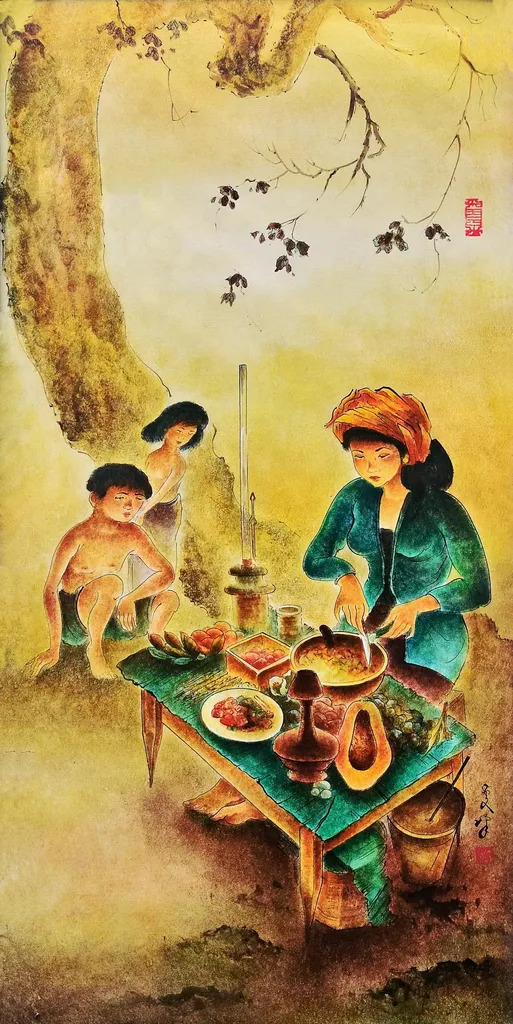This vertically oriented painting, which appears to be influenced by Asian artistic styles—perhaps Japanese or Chinese—is rendered in watercolor on what seems to be manila or scroll-like paper. The background transitions from a predominantly yellow hue at the top to darker browns and black towards the bottom. Centered amidst the backdrop is a tall, curving tree trunk that extends from the middle left upwards, with delicate branches adorned with sparse leaves hanging down.

In the upper left corner, beneath the tree, are two children: a shirtless boy wearing green shorts and a girl, possibly dressed in a light-colored or white dress. The boy sits on a tree stump, and they both appear to be observing the scene in the foreground.

Dominating the foreground is a green-painted wooden table. A woman, seemingly of Asian descent, with long black hair partially covered by an orange or burgundy headscarf, sits behind the table. She wears a green jacket or dress and is engaged in cooking or stirring something in a brown bowl. The table is cluttered with various items, including another dish with vegetables, a square container, possibly a small white plate, and what seems to be a cut-open papaya. The overall composition is delicately painted, lending a light, almost ethereal quality to the scene.